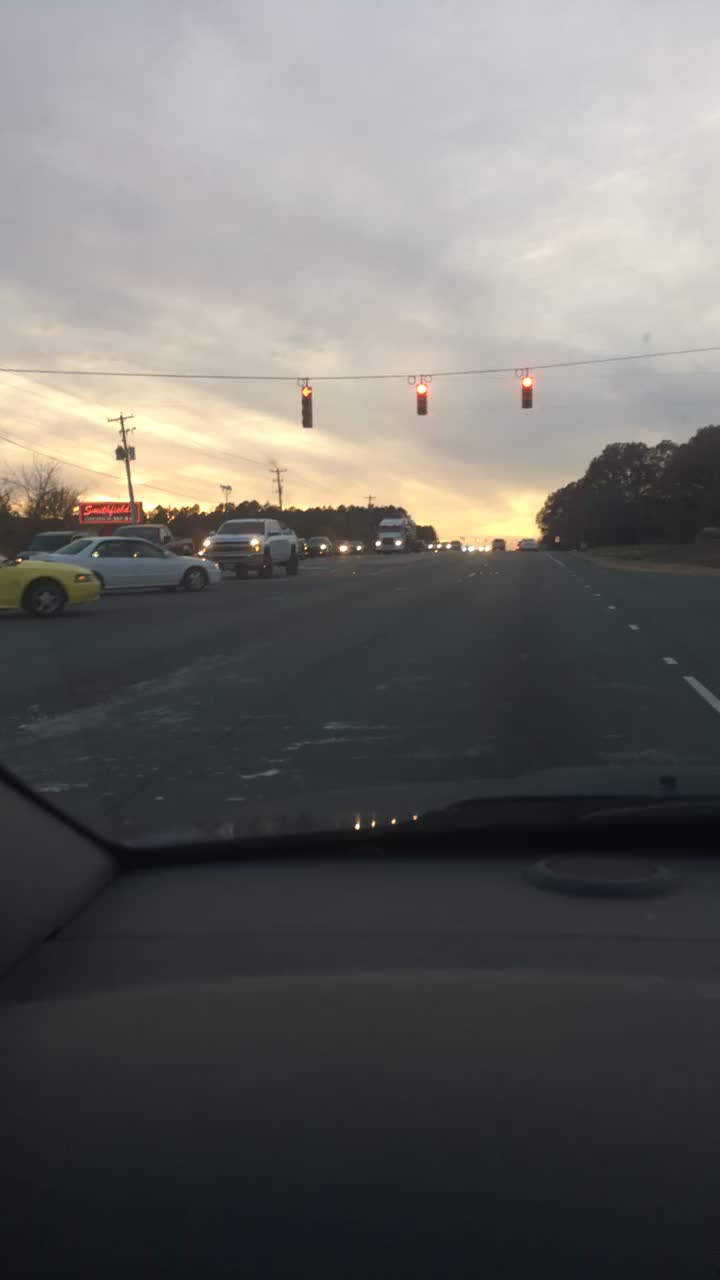A photograph taken with a cell phone from inside a stationary car, either from the driver's seat or the passenger's seat. The image aspect ratio is very tall, capturing mostly the lower half of the car's dashboard and the top half showing a highway where the car is parked at a red light. Indicated by the city traffic lights visible above the road, the lights are red, including two circular red lights and a red arrow. No cars are directly in front of the photographer, but the oncoming lane to the left is busy with various vehicles including a yellow car, a white sedan, a white pickup truck, and a red pickup truck. The sky is a mix of gray clouds with a bright, yellow-orange horizon, indicating it is dusk. On the far left, there are trees—some with leaves and some bare—and a rectangular red Smithfield sign, likely a fast food restaurant. The scene includes lanes marked on the road, and several cars have their headlights on, contributing to the twilight atmosphere.